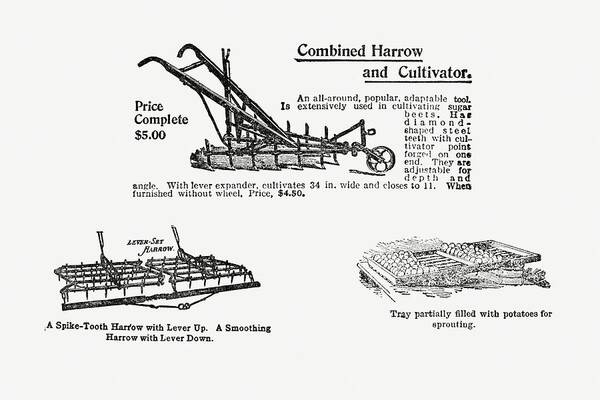This black-and-white image, possibly from an old magazine or newspaper advertisement from the late 1800s or early 1900s, features detailed technical drawings and descriptions of farming implements. The title "Combined Harrow and Cultivator" is prominently displayed at the top of the page. The primary drawing portrays a device with a wheel connected to a triangular frame and handlebars, resembling an old-fashioned lawnmower. This machine features adjustable, diamond-shaped steel teeth with a cultivator point designed for cultivating sugar beets and other crops. Priced complete at $5.00, without the wheel it costs $4.50.

Below this main image, the advertisement includes two additional illustrations. On the left, there’s the "Spike Tooth Harrow with Lever Up" and the "Smoothing Harrow with Lever Down," both depicted with detailed grates and handles. On the right, a tray partially filled with potatoes for sprouting is showcased, further indicating its agricultural utility. This advertisement reflects the old-time marketing style, emphasizing the equipment's utility and adaptability for farmers.